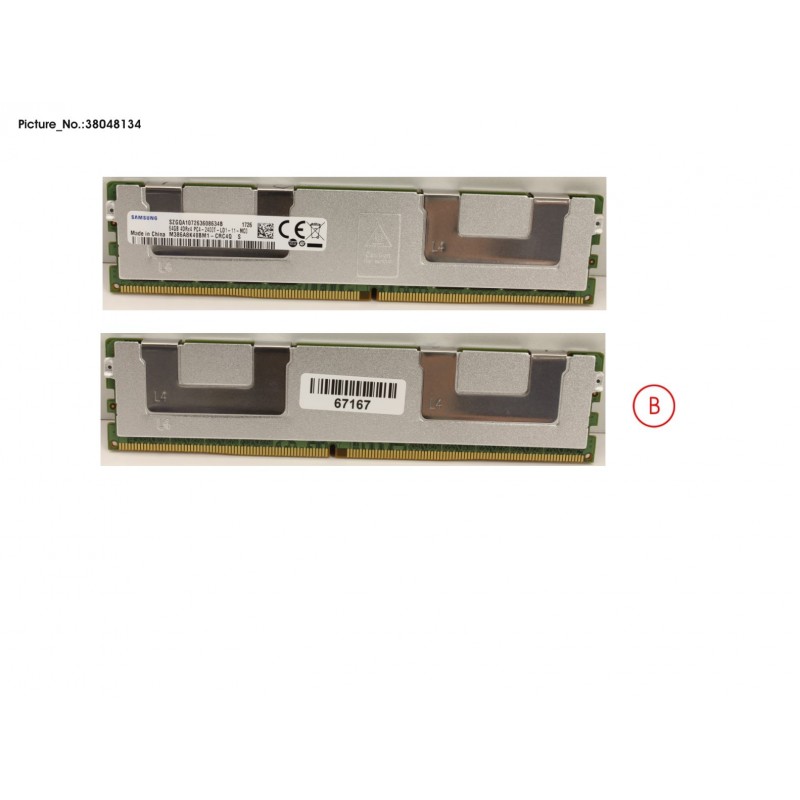The image displays two views of a single RAM stick, a crucial component of a computer's memory system. The RAM stick is a thin, rectangular module reminiscent of the shape of a comb with fine teeth, typically used by men. Each view in the image highlights the array of individual pins designed for connecting to the motherboard. The top and bottom parts of the image seem to show different sides of the same RAM stick rather than two separate memory modules. This is evident from the slight offset of the notch located at the bottom of the connector area, which aligns differently on each side of the single stick. RAM, or random access memory, is essential in computer systems for facilitating quick data access and boosting overall performance.